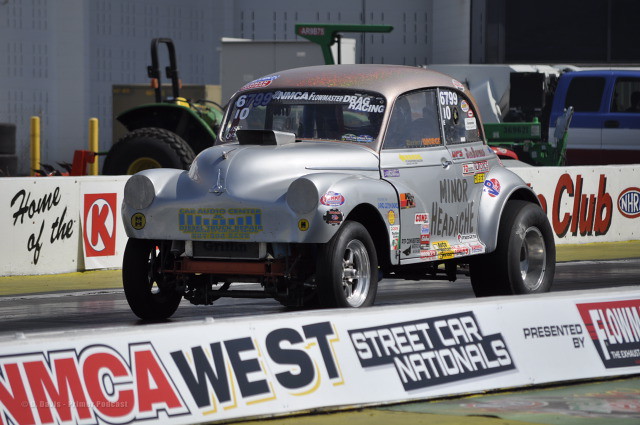The image features a silver, souped-up Volkswagen Bug with exceptionally wide tires, prominently parked on a racetrack. The car, named "Minor Headache," is adorned with various advertisements and stickers, including notable mentions of "NMCA Drag Racing" and "Streetcar Nationals," signaling its racing intentions. The car's front end is devoid of a bumper and headlights, revealing bare metal and a box over the hood, likely for engine ventilation. Its hood is distinctively gold, blending subtly with its silver body unless inspected closely. Behind "Minor Headache," the racetrack scene includes a pair of green John Deere tractors parked side by side and a two-tone blue and white Ford pickup truck, adding to the colorful and dynamic atmosphere of the event.